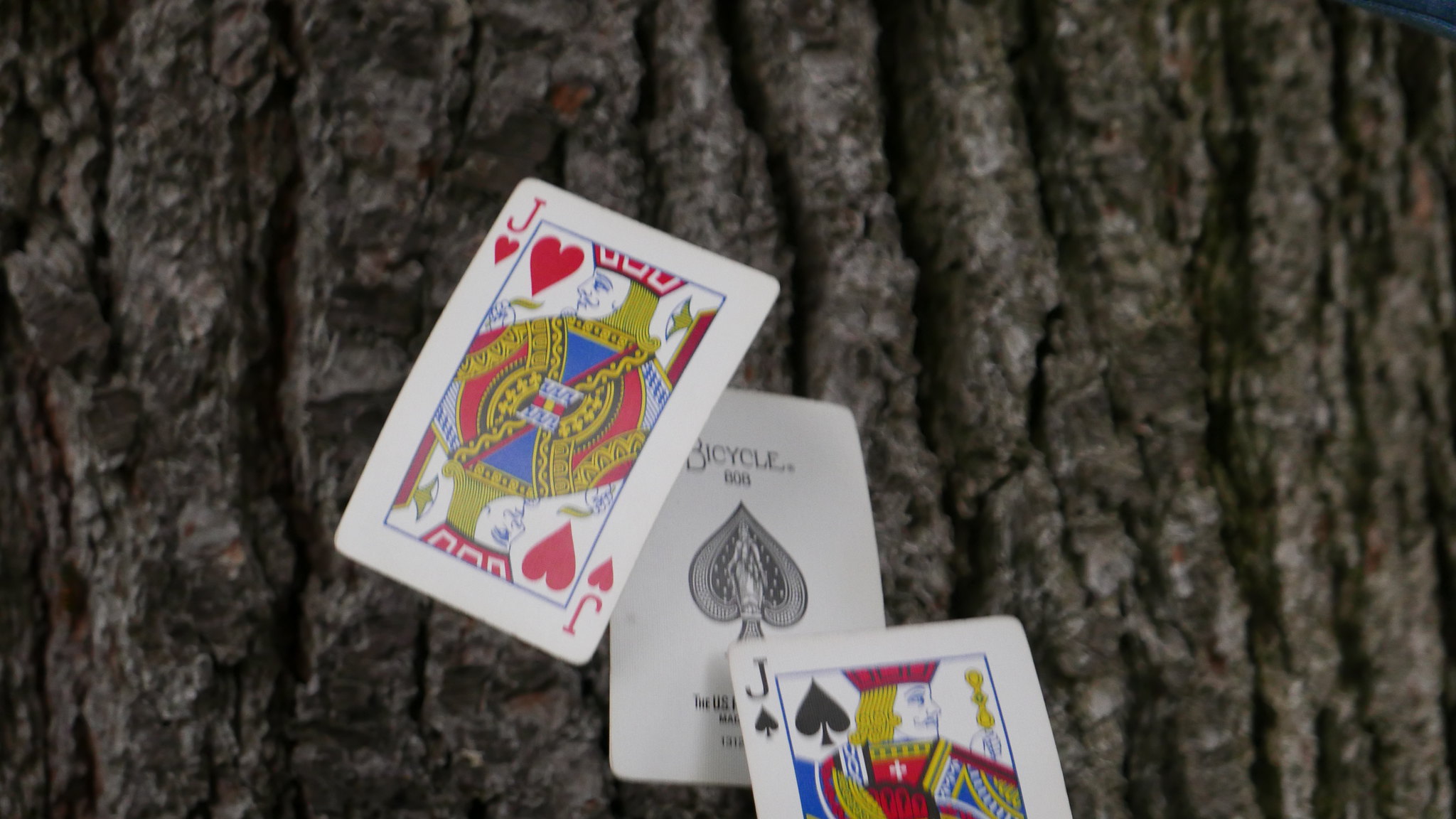The photograph captures a slightly blurry image of three playing cards from a deck, arranged on a surface that resembles tree bark. This bark-like surface features shades of brown, dark gray, and hints of white. The first card displayed is the Jack of Hearts, adorned with red hearts and depicting a figure robed in red, gold, and blue, wearing a red hat with blonde hair. Beneath it lies a card branded with "Bicycle" in black font, showcasing an image of a robed figure in black. The final card in the stack is the Jack of Spades, highlighting a jack and black spade. The figure on this card, similar in attire to the Jack of Hearts, is dressed in blue, yellow, and red robes, with a blonde-haired character donning a red hat and holding a golden scepter-like object.